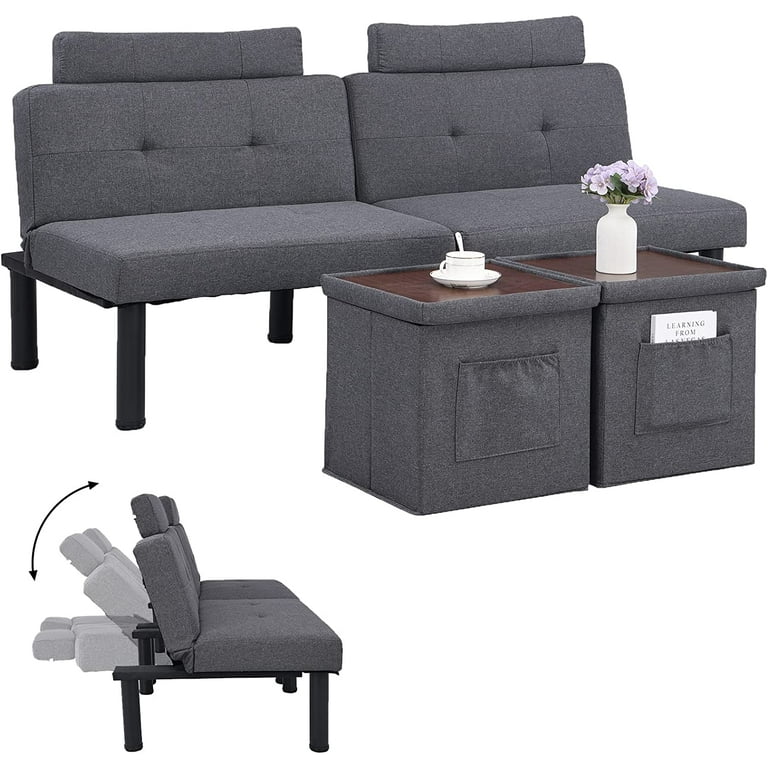This image features a sleek, multifunctional piece of furniture—a gray loveseat without arms, upholstered in dark gray fabric and supported by six black legs. On either end of the loveseat, there are long, cylindrical pillows serving as headrests. The loveseat is shown in a reclining position, suggesting that it can be converted into a bed-like structure, similar to a futon.

In front of the loveseat, there are two small tables. The table on the left holds a white coffee cup with a saucer, while the table on the right features a vintage-style white milk bottle vase filled with purple flowers. Both tables appear to have brown wooden tops and are covered in fabric, with pockets on the front. A book titled "Learning From" is partially visible, tucked into one of these pockets.

The background and setup of the photo give it a commercial feel, as though it's part of an advertisement for this versatile loveseat. The overall design and arrangement suggest a modern and functional living space, suitable for various uses.